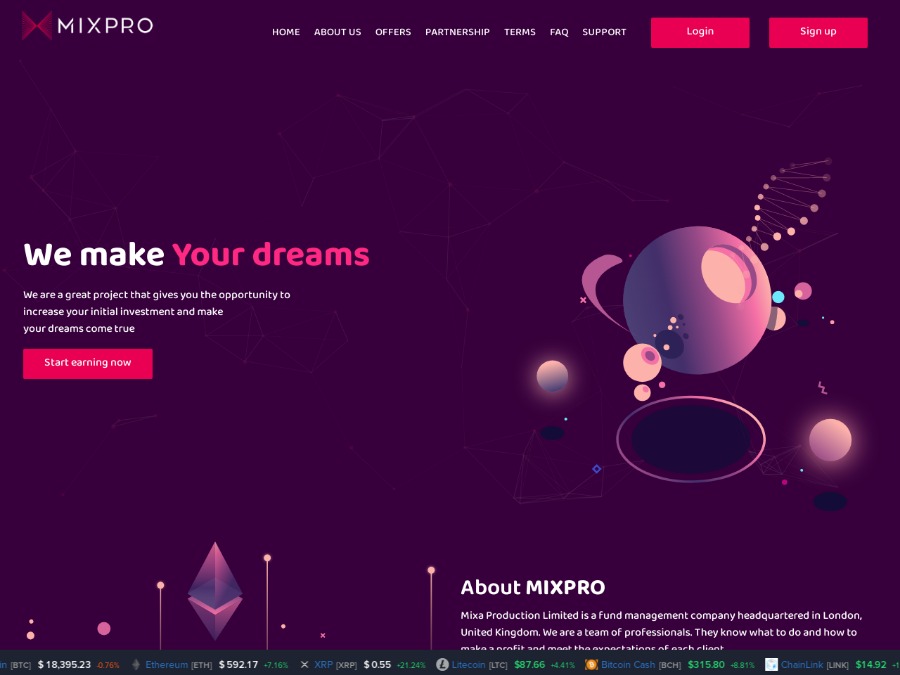This is a detailed description of an advertisement page for Mix Pro, categorized under websites. The background is a deep, rich purple, which sets a striking tone for the content. In the top left corner, the Mix Pro logo is prominently displayed, featuring the brand name alongside a graphic resembling two butterfly wings coming together.

Spanning across the top of the page in white text, the navigation menu includes the options: Home, About Us, Offers, Partnership, Terms, FAQ, and Support. To the right side of this menu, there are two red buttons labeled "Login" and "Sign Up" in white letters.

On the left-hand side, beneath the navigation menu, a tagline reads: "We Make Your Dreams." The text is split into two colors for emphasis—"We Make" is in white letters and "Your Dreams" is in pink. Following this tagline, the site description elaborates: "We are a great project that gives you the opportunity to increase your initial investment and make your dreams come true." Below this, a call-to-action button urges visitors to "Start Earning Now."

On the right side of this section, a captivating, futuristic graphic depicts a series of planets and cosmic elements. One prominent purple planet features a radiant white light at its center. Among these celestial bodies, a 3D structure resembling a DNA helix floats, adding a scientific allure to the design.

At the bottom of the page, a section titled "About Mix Pro" offers additional information about the project, inviting users to delve deeper into the platform’s offerings.